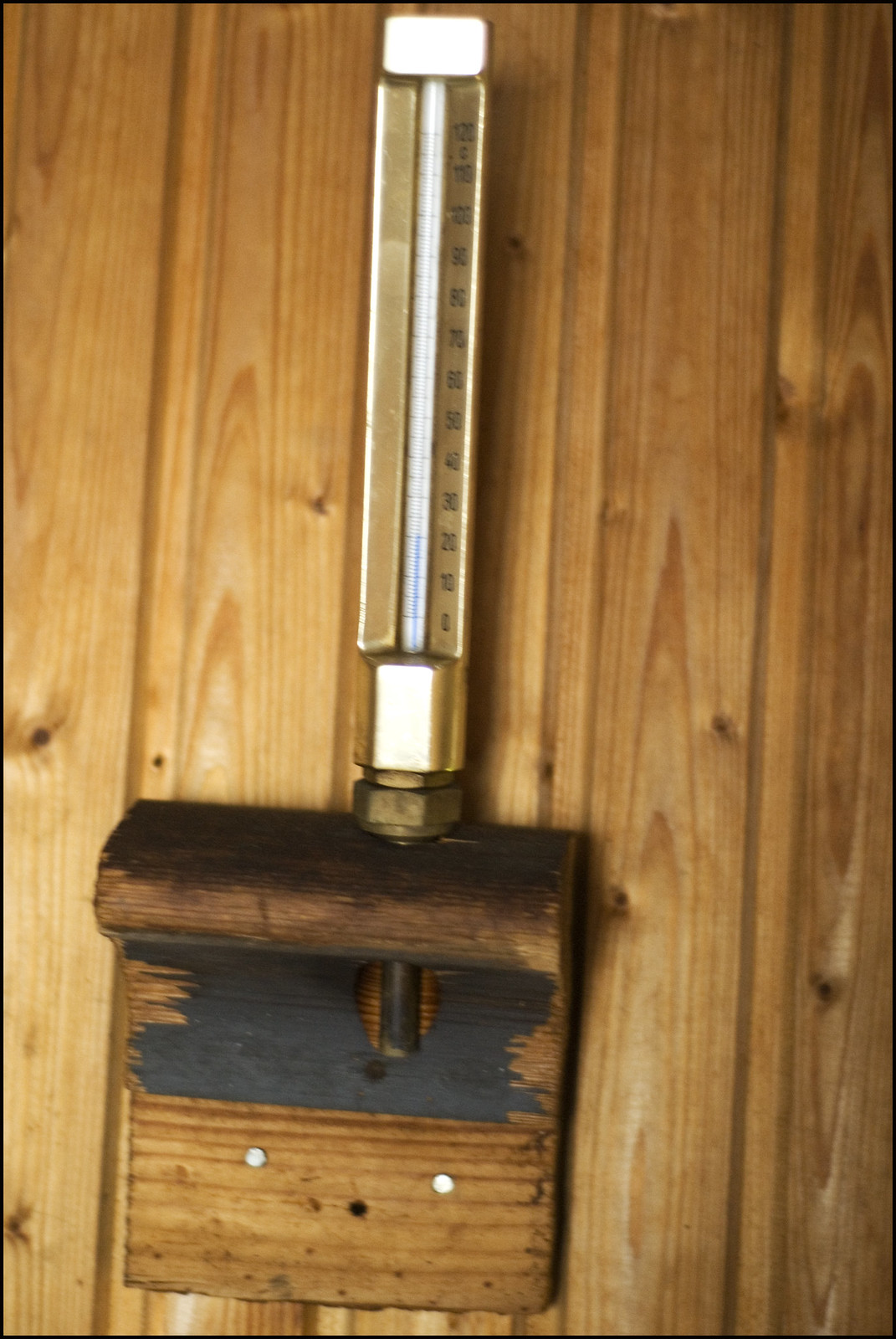The photograph features a retro thermostat, securely mounted onto a light brown wooden wall. The thermostat exudes a vintage charm with its brassy, gold-toned frame that elegantly encases the device. The central section of the thermostat, which houses a vertical temperature indicator, is a crisp white, creating a striking contrast. This indicator is further highlighted by a blue bar that moves up and down to display the current temperature. Positioned just below the thermostat, there is a matching wooden piece, seamlessly blending with the background and completing the nostalgic aesthetic of the scene.